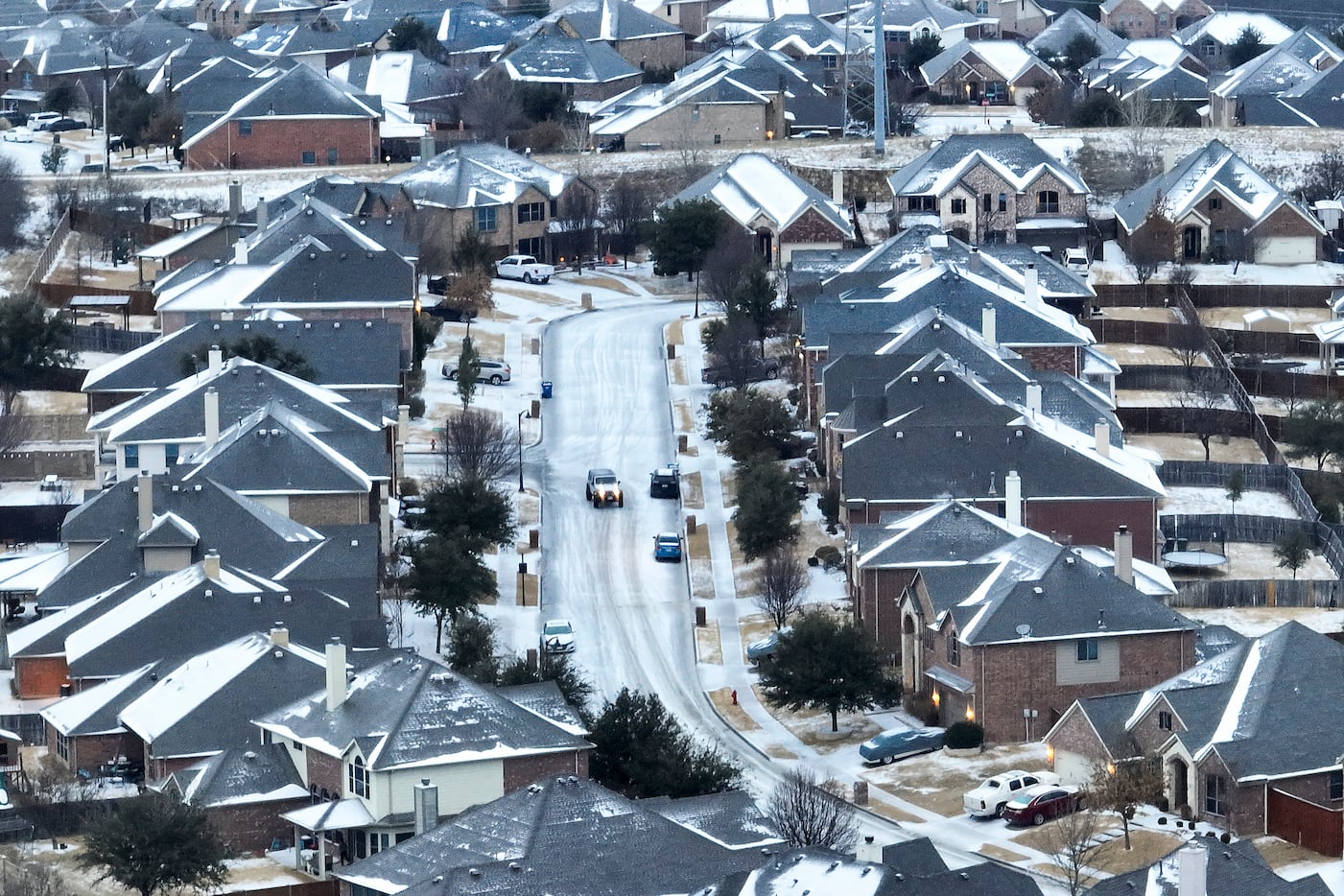This aerial shot, likely taken from a drone, captures a residential neighborhood blanketed with a recent dusting of snow. The scene features numerous houses closely nestled together, resembling expensive tract homes, many of which are two stories high with gray roofs partially covered in snow. A central, curving main road slices through the image, flanked by mailboxes at the curbs and dotted with vehicles. Notably, a white SUV with yellow-tinted headlights can be seen driving down this road, reflecting the snow's cold ambiance. Numerous cars are parked in driveways and alongside the street, but there are no people visible. The backyards of the houses are fenced off, with wooden fences separating each snowy yard. Scattered trees in the front yards and a consistent layer of snow on both the ground and the rooftops emphasize the chilly, wintry day in this crowded subdivision.